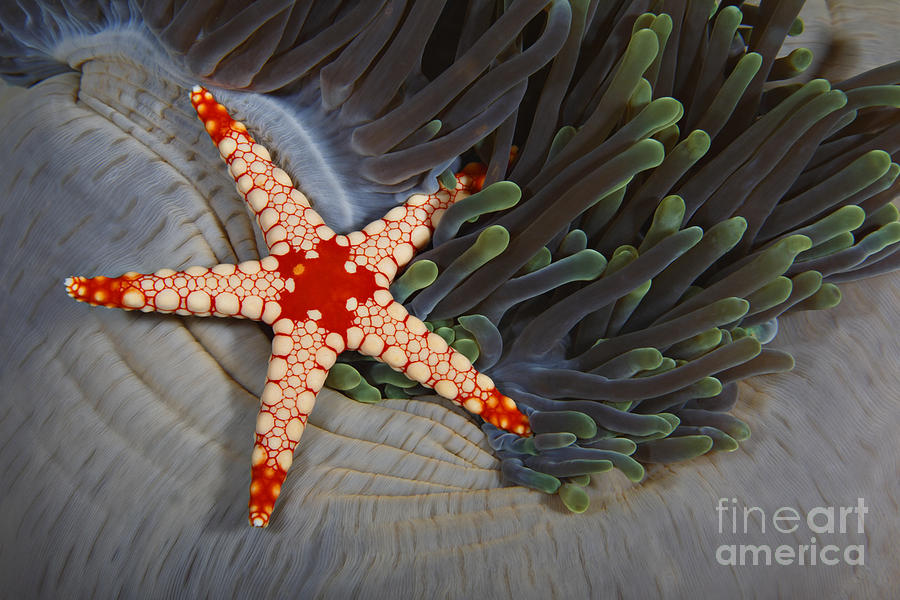The image is a highly realistic 3D render depicting an underwater scene with a vibrant starfish positioned slightly to the left of center. The starfish, characterized by its bright red, nearly orange tips, has a vivid red center resembling a pentagon or octagon shape. Its legs display a series of white bumps along their length, interspersed with reddish-orange areas. The starfish rests on a striking, white coral bed that appears thread-like in structure. To the right of the starfish, green sea anemone tentacles or similar fluorescent tentacles wave gracefully in the water, accompanied by grayish tentacles extending from above. This detailed, lifelike scene is underscored by a watermark in the bottom right corner that reads "Fine Art America" in transparent text.